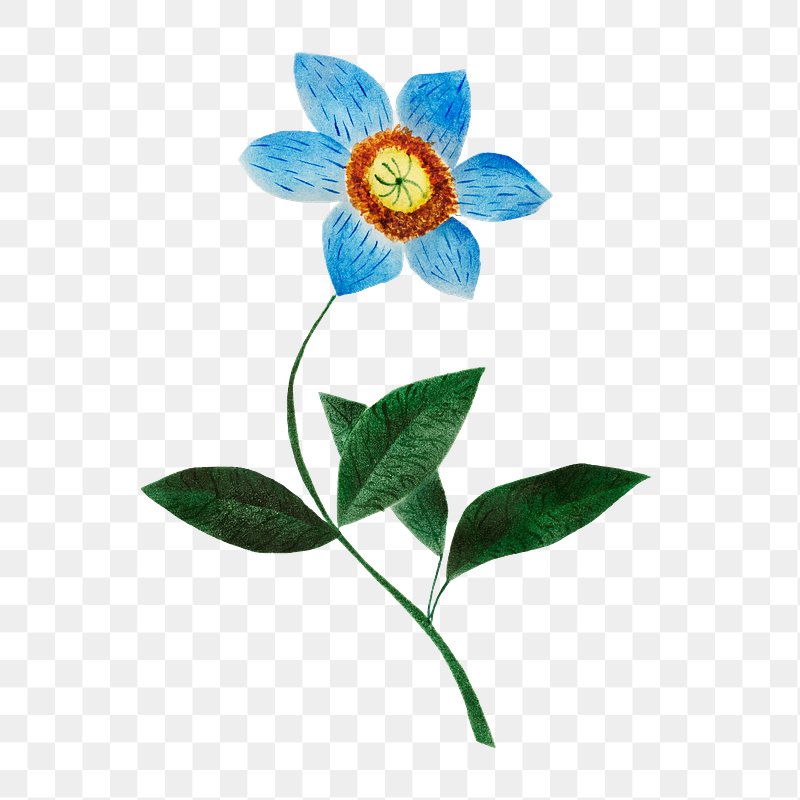This detailed drawing or painting depicts a vibrant blue flower against a subtle gray and white checkered background. The background's checkerboard design, with its small squares, provides a gentle contrast that highlights the central floral subject. Positioned centrally, the flower features a green stem with two medium-sized, pointy leaves branching off to the right, and farther up, another set of leaves — one extending to the left and one to the right. The leaves are a rich, dark green, akin to ivy. 

At the top, the flower blooms with six light to medium blue petals, each detailed with darker blue streaks. The petals surround a distinctive center composed of a rough-textured brown ring filled with fibrous details. Inside this ring, a yellow core is accentuated with a green star-like pattern, featuring eight green lines radiating outward. The entire composition is meticulously clear, benefiting from bright natural lighting that enhances its vivid colors and intricate details.